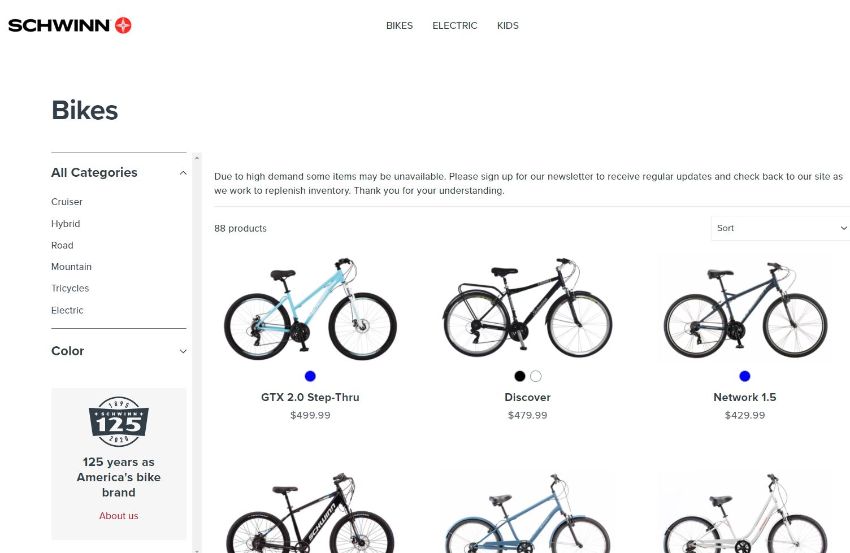This image is of the Schwinn homepage dedicated to bikes. In the upper left-hand corner, the "Schwinn" logo is prominently displayed in bold black font. Adjacent to it, there is a red circular symbol featuring a white cross at its center.

Across the top-center section of the page, there are three navigational links labeled "Bikes," "Electric," and "Kids." On the left side of the page, there's a larger, bolded "Bikes" heading in black font, separated by a thin gray line. Below, "All Categories" is also bolded, followed by a list of bike types: "Cruiser," "Hybrid," "Road," "Mountain," "Tricycles," and "Electric."

Further down, a new section starts with the word "Color" accompanied by a dropdown arrow on its right. Below this, there’s a small box featuring the number "125" alongside the phrase "125 years as America's bike brand," celebrating Schwinn's longevity. 

In the central area of the page, six bikes are displayed with their respective prices. These bikes appear to be of different models but are all mountain bikes.